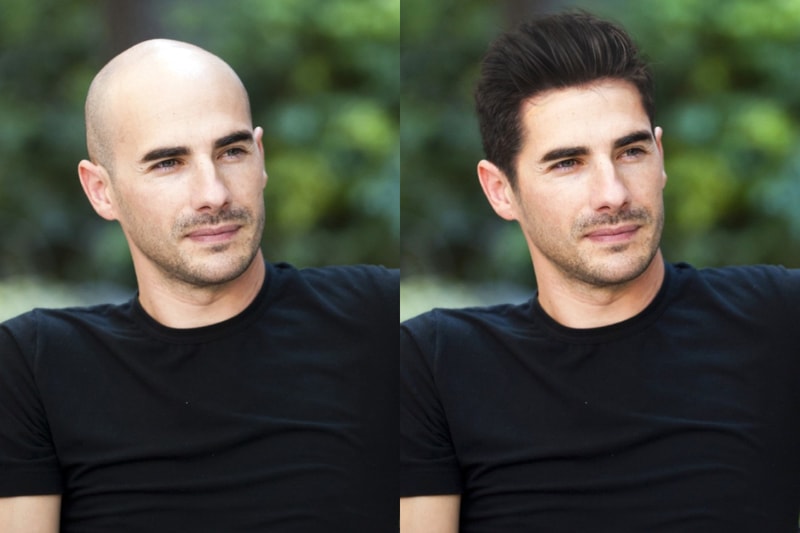The image features two side-by-side photos of the same man in identical poses, both showing him from the chest up against a backdrop of green leaves. The primary difference between the photos is the man's hairstyle. In the left photo, he is bald with a light mustache, while in the right photo, he has a full head of brown hair styled back and a heavier mustache accompanied by a five o'clock shadow. In both photos, he wears a black t-shirt and has thick eyebrows. The images are likely photoshopped to highlight the contrasting hairstyles. The overall setting is bright with clear visibility and vibrant colors.